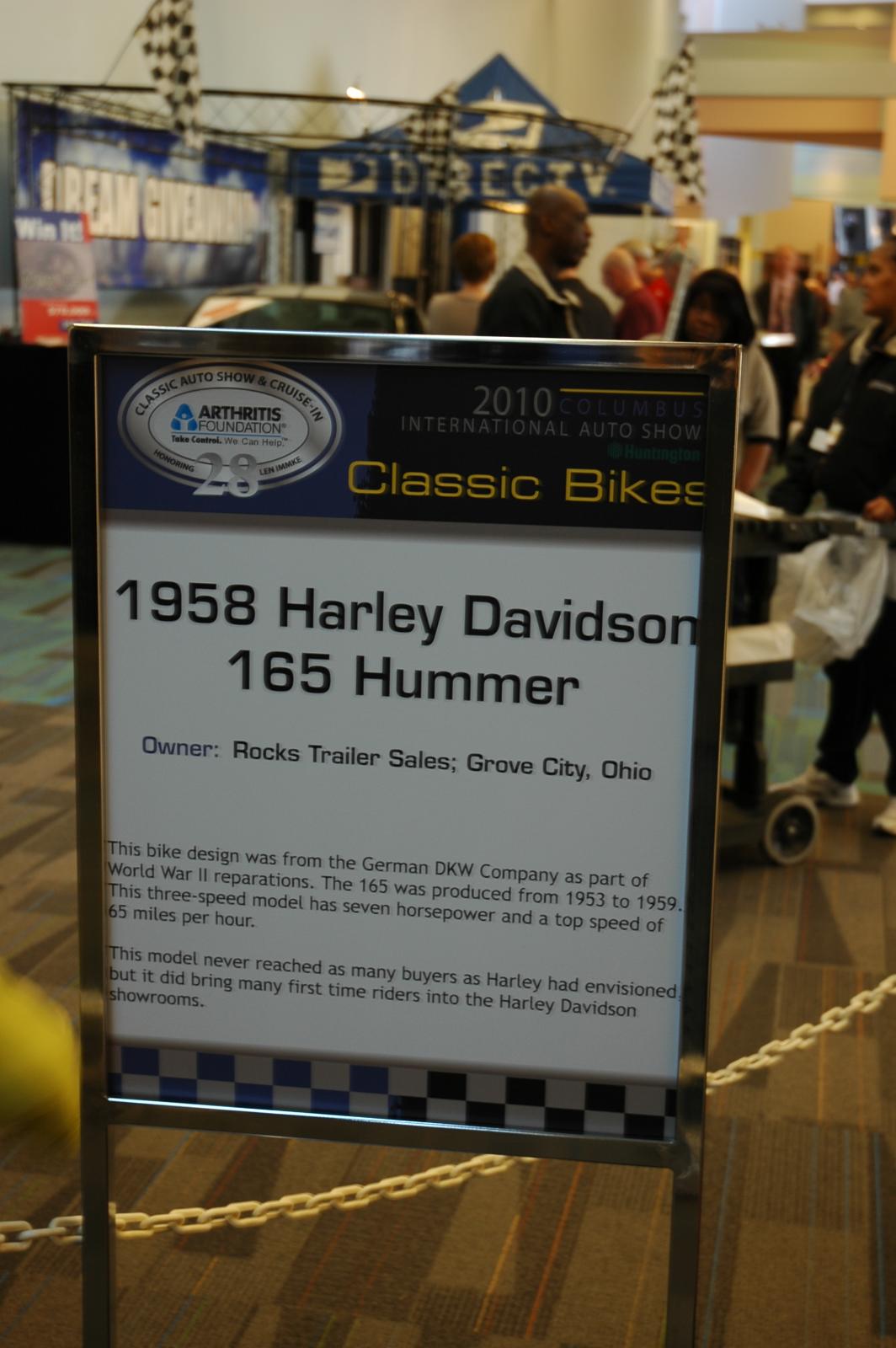The photograph features a sign prominently displayed at the 2010 Columbus International Auto Show, specifically in the Classic Bikes section. The sign, which has a white background bordered by silver metal and a checkered flag design at the bottom, provides detailed information about a 1958 Harley-Davidson 165 Hummer. This motorcycle, owned by Rocks Trailer Sales from Grove City, Ohio, is noted for its design origins from the German DKW company during World War II reparations. Produced between 1953 and 1959, the 165 Hummer is a three-speed model with seven horsepower and a top speed of 65 miles per hour. Though it fell short of Harley-Davidson's sales expectations, it succeeded in attracting many first-time riders to their showrooms. The scene behind the sign is a busy auto show setting, with a blurred background featuring numerous attendees, DirecTV branding, and Dream Giveaway signs, all contributing to the lively atmosphere characterized by hues of blue and white.